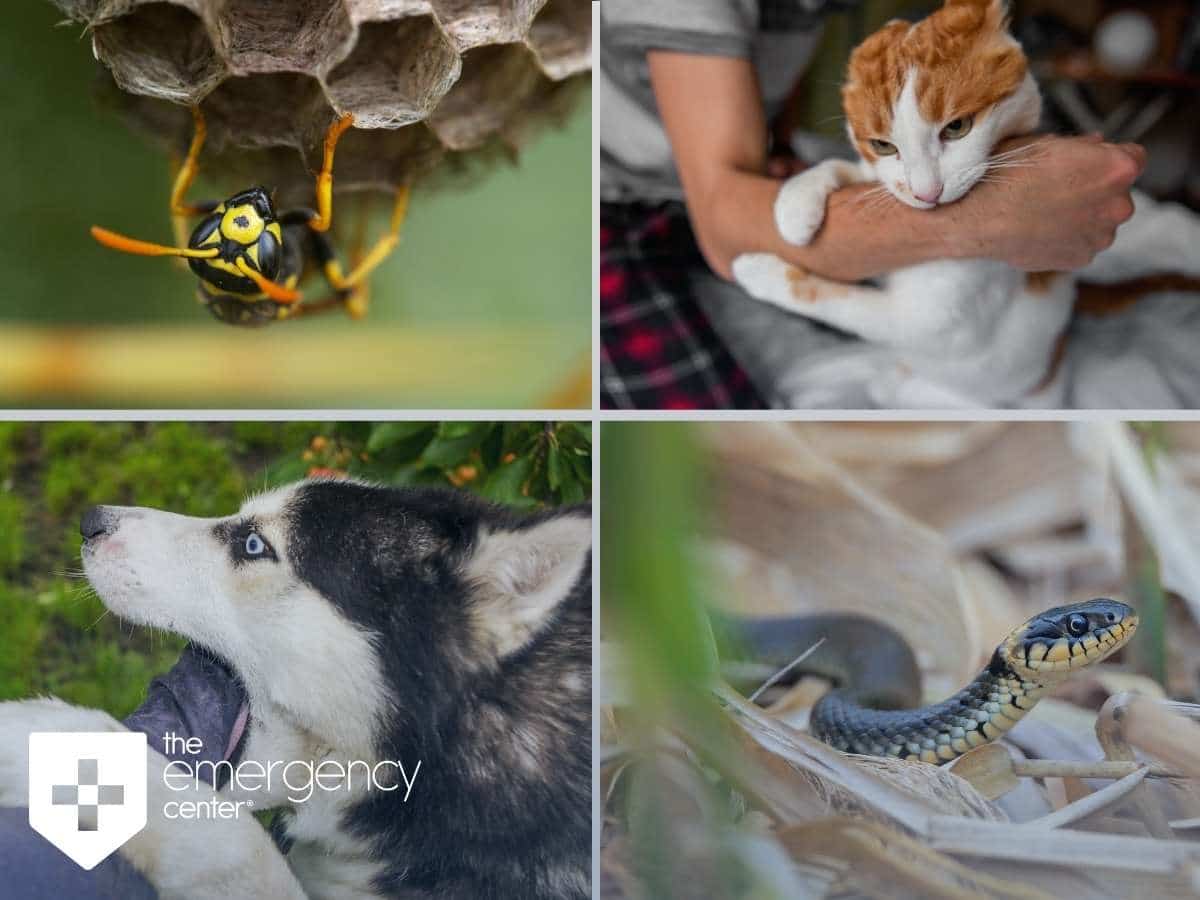This composite image is segmented into four quadrants, each featuring a different animal. The top left quadrant showcases a wasp hanging upside down from a partially constructed paper nest, identifiable by its distinctive yellow and black coloration. In the top right quadrant, a person is holding a cat that is playfully gnawing on their arm; the cat has an orange head, a white face, and a predominantly white body with a few orange spots. The bottom left quadrant portrays a black and white husky dog with striking blue eyes, chewing on a bone. The bottom right quadrant presents a snake slithering out from a grassy area, characterized by its dark scales and yellowish body. Notably, the lower left corner of the image contains the text "the emergency center."